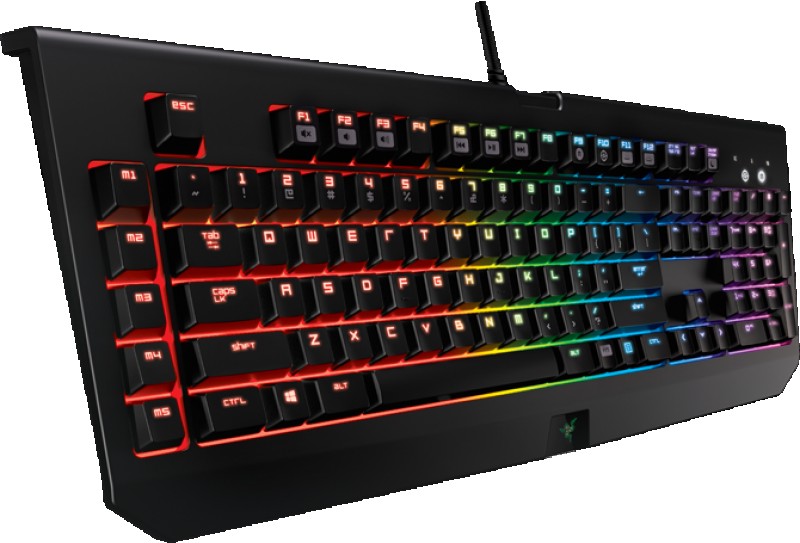The image showcases a mechanical keyboard, well-centered but angled diagonally, with the left side closer and the right side further away. The keyboard is entirely black with illuminated keys that display a gradient of colors from left to right: beginning with red and orange, transitioning into yellow and green, and finally into blue, turquoise, and purple. Each key's label is visible, and there's a number pad prominently on the far right side, lit up in purple. The background appears to have been photoshopped out, leaving it stark white. A black cord or antenna protrudes from the middle top of the keyboard about an inch high, adding a subtle detail to the overall sleek, vibrant aesthetic. This image, devoid of any additional text, seems perfect for either an online sale listing or a social media post showcasing the keyboard.